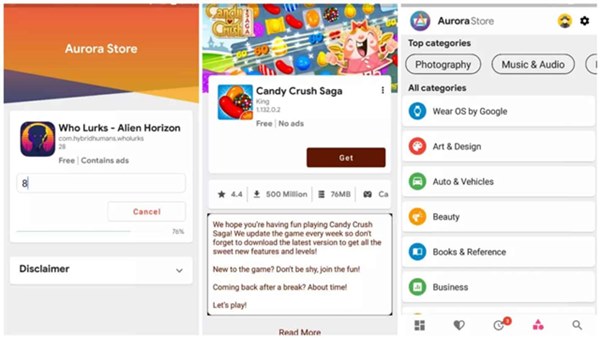The photo showcases a mobile phone screen displaying an account interface linked to a gaming app store, segmented into three separate but continuous portrait-oriented screenshots arranged side by side to create a larger landscape view. 

On the leftmost screenshot, the screen introduces the "Aurora Store" in white font against an orange background shaped like a rhombus or trapezoid, intersecting with a purple square. Below, a gray background features a white box, highlighting a game called "Who Lurks Alien Horizon" labeled as free and containing ads.

The central screenshot focuses on another game featured in the Aurora Store. It presents a white box displaying the "Candy Crush Saga" icon, accompanied by its name. Beneath it, a red rectangular button with white text reads "Get," presumably to download the game.

The rightmost screenshot provides a broader view of the Aurora Store interface. At the top left corner, the store’s logo is shown, resembling a shopping bag. Adjacent to it, a circular avatar icon and a gear icon for settings appear. Below these icons, a gray box labeled "Top Categories" and another "All Categories" prompt further exploration. Various sub-categories follow underneath, including options like "Wear OS by Google," "Art and Design," and "Auto and Vehicles," each paired with respective icons.